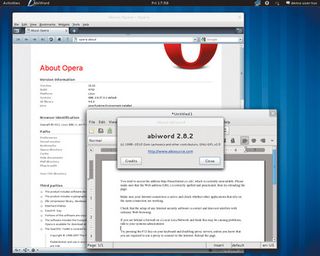In this image, a MacBook screen displays an open browser page highlighting information about the Opera web browser. Various modern dialog boxes are visible, showcasing sleek and contemporary design elements. The background of the webpage is primarily blue, complemented by white, black, and red accents that add visual contrast and emphasis to specific elements on the screen. The MacBook itself is set against a neutral backdrop, allowing the vibrant colors and details of the browser page to stand out prominently.